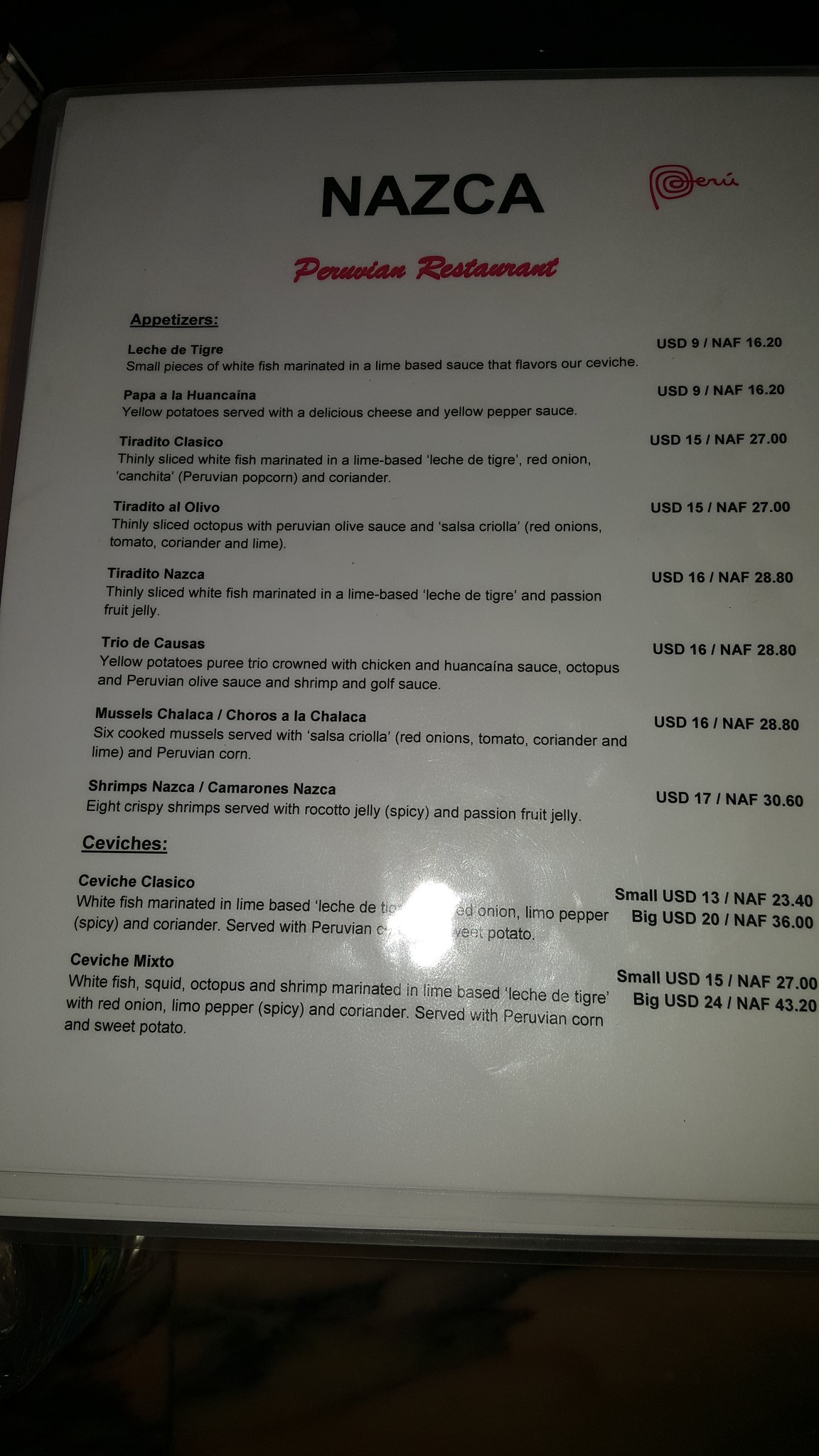This image features a menu from a restaurant named Nazca, prominently displayed at the top of the menu in black text on a white background. Directly underneath "Nazca," there is a word in red starting with the letter "P," possibly "Parisian," followed by the word "restaurant." The menu is presented with two underlined categories; however, the text is small and difficult to discern. The first category contains eight menu items, while the second category, which appears to be titled "Services," lists two offerings. The menu appears to be laminated, as indicated by a noticeable reflection of light in the center bottom area, particularly over the description of the first service offering.